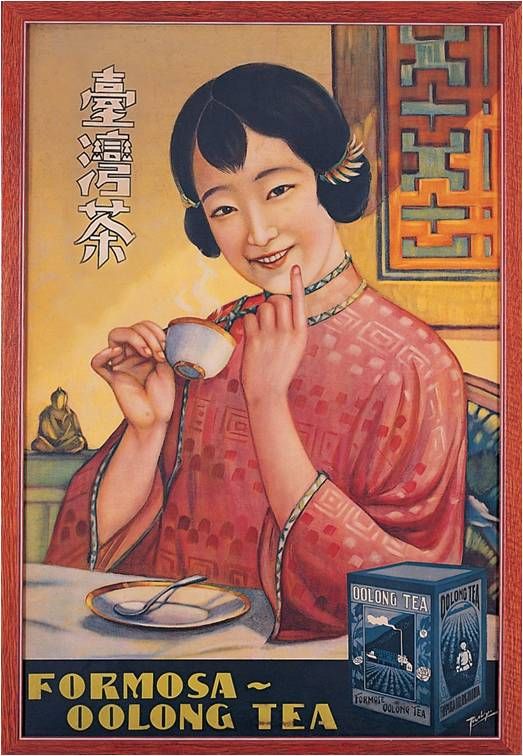The image is a detailed, colorful advertisement featuring a young Chinese woman, possibly in her 30s, enjoying a cup of Formosa Oolong Tea in what appears to be her home. She wears a pink dress with a pattern of squares and dots, reminiscent of traditional Chinese attire, and her hair is styled in two side buns. Seated at a table with a white tablecloth, she gracefully holds up a white teacup with her right hand, while her left hand rests thoughtfully against her chin as she smiles. Below her on the table, there is a matching saucer and a spoon. To the left of the woman, vertical Chinese text is visible beside her head, and a small Buddha statue is situated on the countertop. On the right side of the image, the background features yellow walls and a window with intricate openings, indicating an indoor setting. At the bottom of the illustration, the text "Formosa Oolong Tea" is prominently displayed alongside a blue box of the tea. The artist's signature is located in the bottom right corner of the poster.